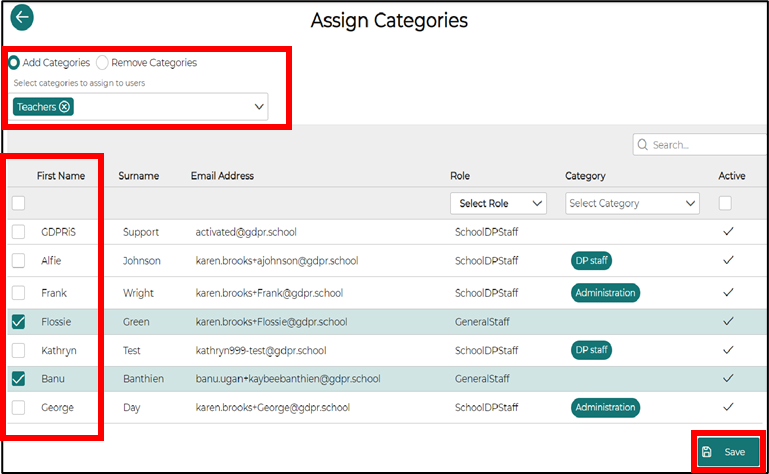The image is a screenshot captured in portrait mode with a thin black border encasing it. Various sections are emphasized by red highlights. At the upper left corner, a green "backwards" button is easily noticeable. The upper center of the image features the heading "Assign Categories."

Below this heading, the first highlighted area is a form for managing categories. You can either add or remove categories, with the "Add Categories" button prominently displayed in green. This section instructs users to "Select categories to assign to users," where "Teachers" have been added via a green text entry.

Within this form, there's a highlighted drop-down menu situated amidst several column headers, which include "First Name," "Surname," "Email Address," "Role," and "Category Active." The "First Name" column is highlighted in red, drawing attention to the listed names: G.D. Priss, Alfie, Frank, and Flossie—all of which have green checkmarks next to them, indicating their selection. Katherine Banu and George are also highlighted, rounding out the first column of names. The remaining columns contain corresponding information such as surnames, email addresses, and roles. There's also a drop-down menu for selecting roles and categories, with options like "DP staff administration."

At the bottom right corner of the image, a red-highlighted green "Save" button reminds users not to forget to save their changes, completing the detailed navigational guide of the screenshot.